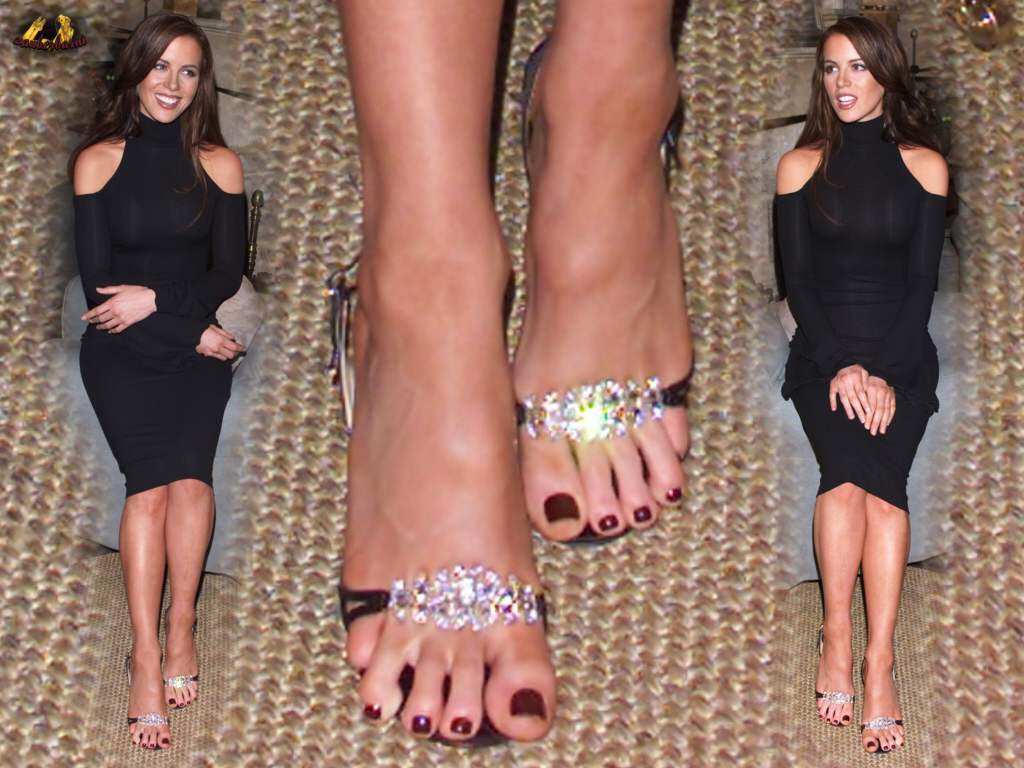This intricate composite image presents a scene set on a tan carpet, where it appears multiple photos have been seamlessly stitched together. On both the left and right sides, we see a young woman with long dark hair extending below her shoulders, dressed in a black dress. She is seated on a chair, potentially at a fashion event held indoors. Both versions of the woman focus on her diverse expressions: her left-side image captures her smiling, with forearms crossed, looking forward and slightly to the right. Conversely, on the right side, she gazes forward and slightly to the left, with her mouth open in a non-smiling expression, and her hands resting palms down on her lap.

Centrally displayed, there's a detailed close-up of her ankles and feet. Her toenails are painted red, and she wears sandals adorned with sparkling sequins over the strap, which glimmers against the subdued backdrop. The image interestingly shifts focus to her feet without any text or clear indicators of time. Additionally, a rounded object, whose details are indistinct, resides in the upper left corner, adding a touch of mystery to the setting. Colors throughout the image include black, tan, brown, gray, silver, and white, maintaining a harmonious but varied palette.